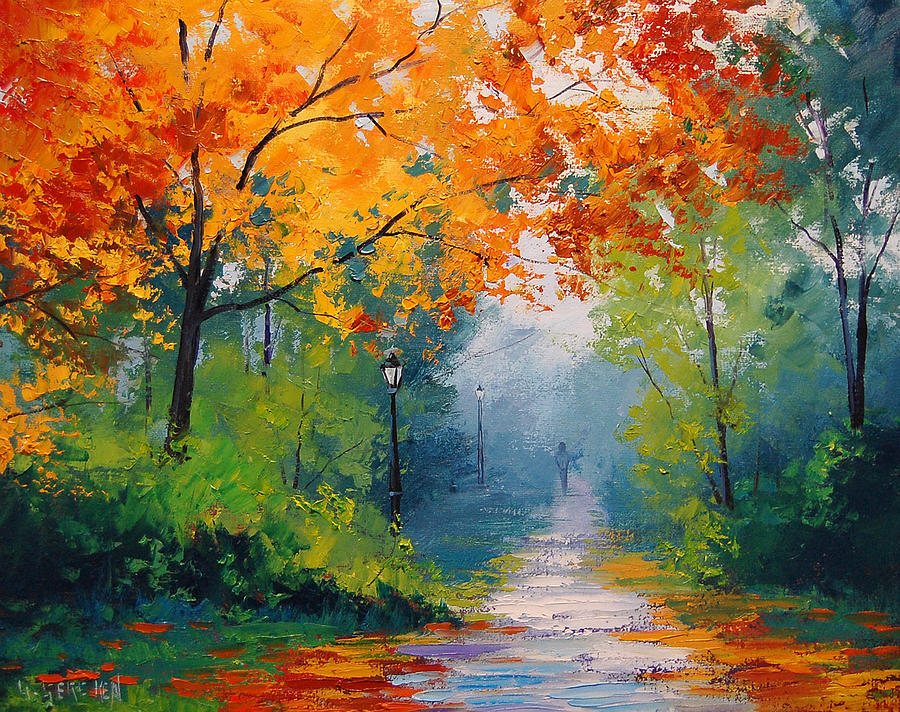This painting depicts an autumnal scene of a park or forest, likely rendered in oil or watercolor. Vibrant and pastely colors dominate the artwork with a mix of green, orange, red, and yellow hues suggesting the fall season. A lone person walks down a white or gray pathway that stretches from the foreground into the distance, flanked by dense forest and trees. The left side features a prominent tree with brilliant orange and red leaves. On the right, trees display lighter greens shading to yellows. Scattered on the ground are fallen leaves, mingling with patches of green shrubbery and hints of red mushrooms. The pathway is lit by black street lamps with white centers, standing to the left of the pathway. The atmosphere is overcast, giving the scene a soft, reflective quality.